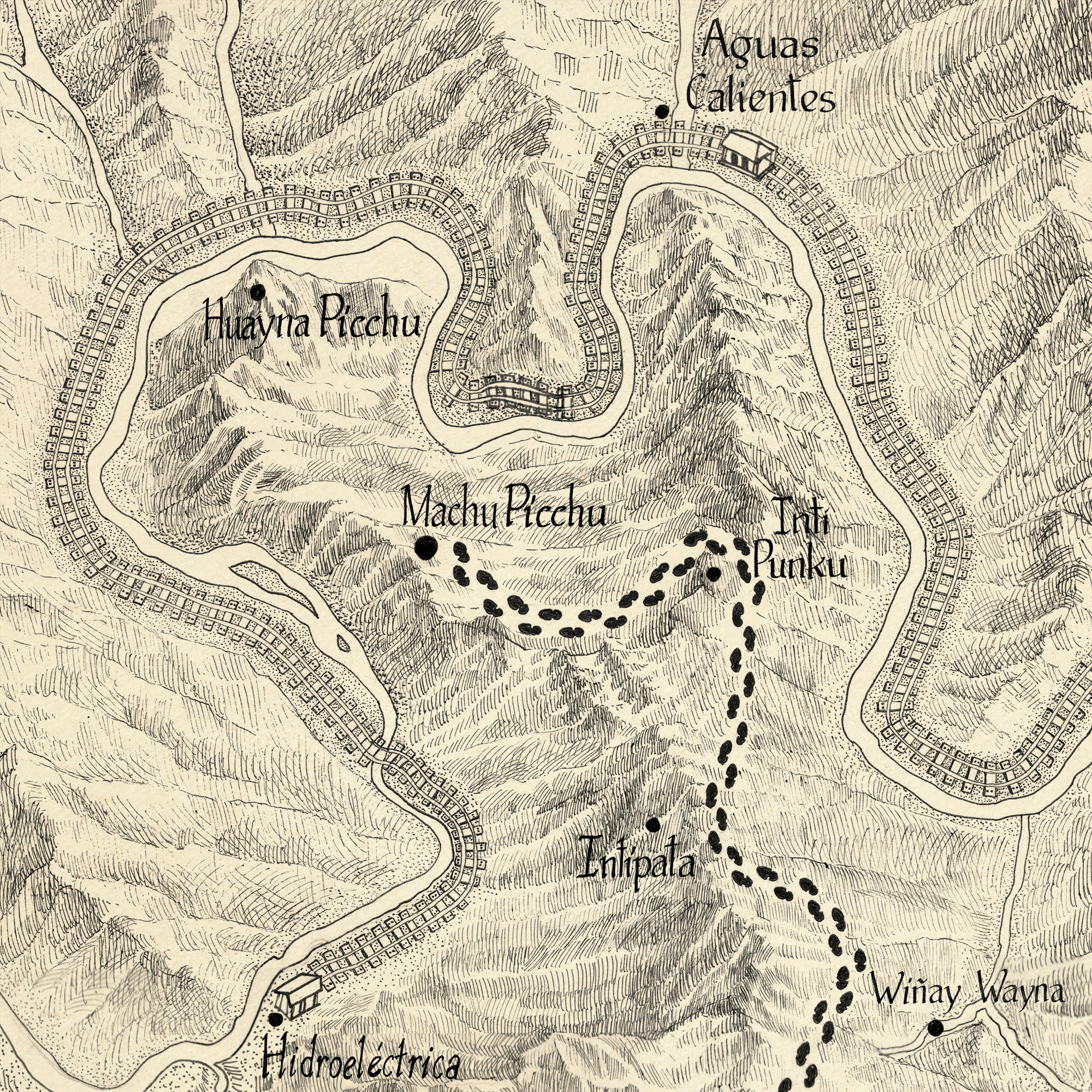The image is a black and sepia-toned traditional rendering of a map with Machu Picchu prominently at the center. Surrounding Machu Picchu on the map, to the northwest is Huayna Picchu, to the northeast is Aguas Calientes, east of Machu Picchu is Antipuco, and south of these locations lies Enlipata. Further, to the southwest, you can find Hidroelectrica, and to the southeast is Huayna.

The map is drawn to resemble a pencil or charcoal sketch on cream-colored or papyrus-like paper, lending it an antique aesthetic. It is marked by several man-made features including detailed winding train tracks that begin at Hidroelectrica, encircling Huayna Picchu and Machu Picchu, and passing near Aguas Calientes before leading off the map. Additionally, a foot trail is illustrated starting from the south near Huayna and Enlipata, stretching up to Intihuanco and culminating at Machu Picchu. The map also highlights mountain ranges, rivers, and streams, effectively shaded in black and gray to give a clear and intricate depiction of the landscape. This map serves as a simplified, traditional contrast to the more modern and complex 3D versions available today.